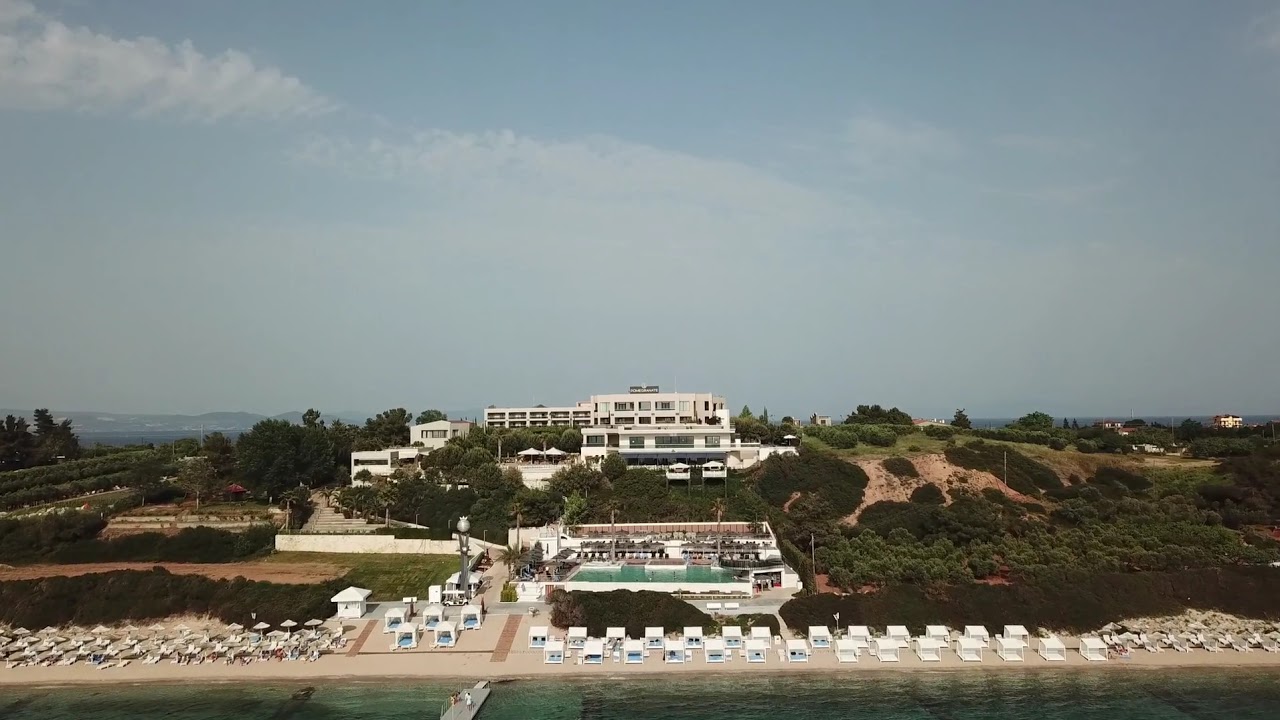This image is a detailed bird's-eye view of a luxurious seaside resort situated on a shore, potentially on a hillside or a small island. At the bottom, we observe a tranquil body of water and a pier extending into it, with some people walking on the dock. The sandy beach adjacent to the water is lined with numerous neatly arranged beach chairs and small white gazebos, some occupied by people enjoying the seaside. Just above this area, there is greenery with trees and bushes, suggesting a natural and serene environment. Further up the hillside, several layers of buildings are visible. The larger white structure, possibly a few stories tall, appears to be a significant resort or hotel. This building might feature additional amenities like a pool. The scene is set under a grayish-blue sky with a thin, transparent cloud cover, giving the sky a slightly gray tone. This well-organized and high-end beach resort evokes a sense of tranquility and elegance, with its vibrant greens, whites, browns, and blues harmoniously blending into the coastal landscape.